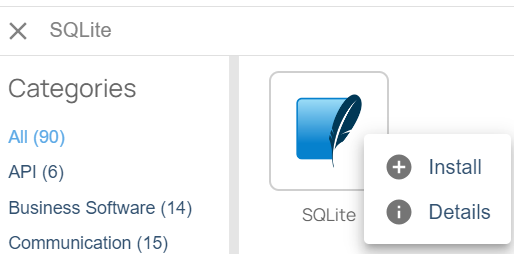This image is a screenshot of a software interface likely displayed on a laptop. Dominating the scene is a window with a white background and light grey text. At the top left corner, there's a conspicuous 'X' for closing the window. Prominently displayed is the title "SQLite," with 'SQ' in uppercase letters.

Below this title, there's a navigation menu labeled "Categories." The default category, indicated as "All (90)," is selected and highlighted with a light baby blue color. Other categories listed include "API (6)," "Business Software (14)," and "Communication (15)."

Additionally, there is an icon featuring a quill and a blue folder, often the representation for SQLite. Adjacent to this icon is the option to "Install" the software, denoted by a plus sign and "Install" text. Beneath it, another plus sign leads to "Details" about the software.

The interface is organized with subtle light grey borders, giving it a clean and structured feel. Beyond these elements, there is no further text or any date stamps visible, leaving out more detailed descriptions or additional context about the application.